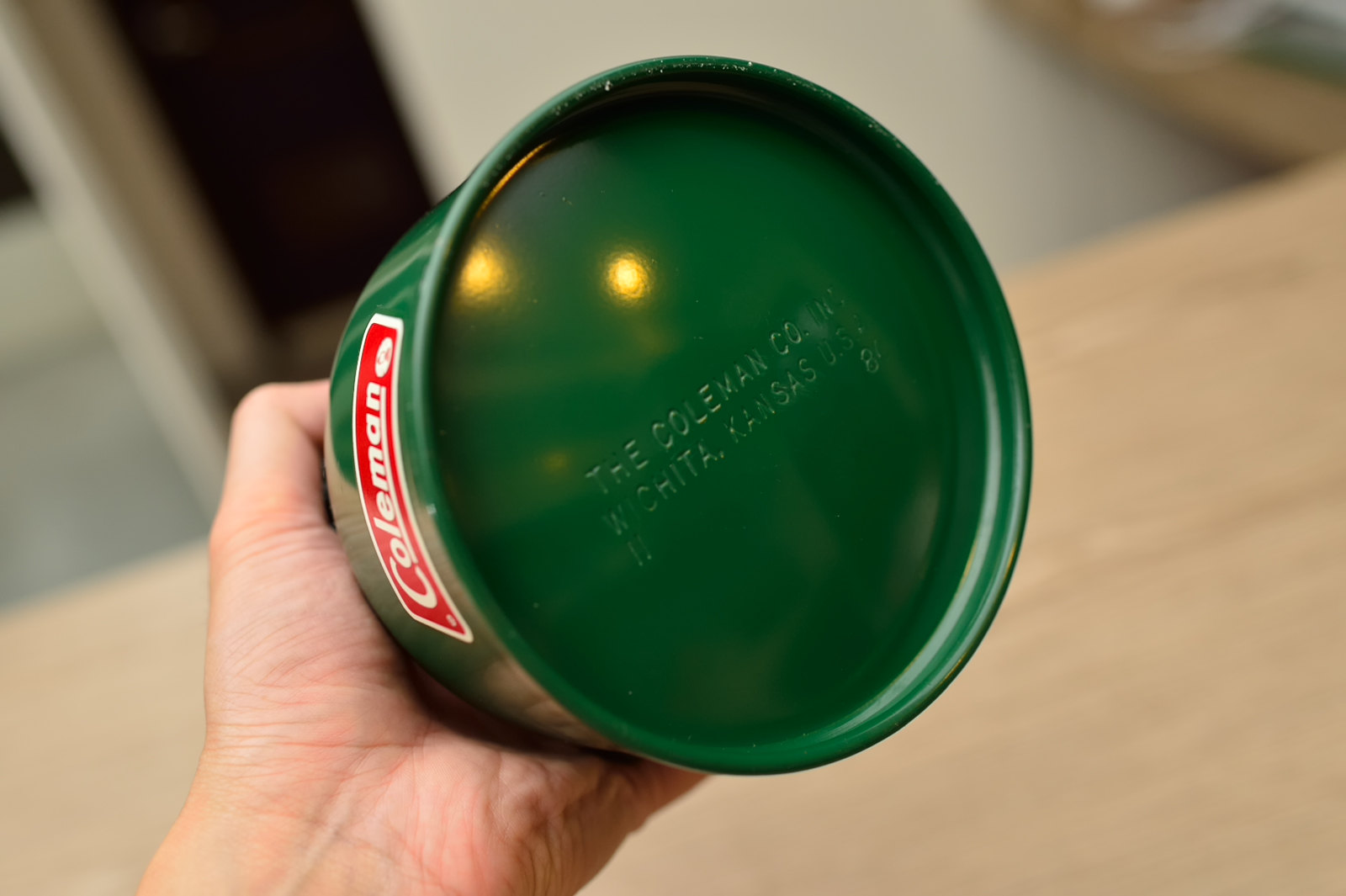A close-up photo showcases a dark green cylinder being held in a person's left hand, which is a light-skinned hand with the thumb at the top and the fingers grasping the lower part of the cylinder. The background is blurred, though there might be a tan table and possibly a gray floor in the out-of-focus area. The focal point, however, is the dark green cylinder which appears brand new, with no visible scratches. Light reflects off its surface, enhancing its fresh appearance. Attached to the cylinder is a white label edged in red, bearing the brand name "Coleman" prominently. Additional text on the label suggests the product is associated with the Coleman company, headquartered in Wichita, Kansas, USA, although the details below the brand name are somewhat unclear.